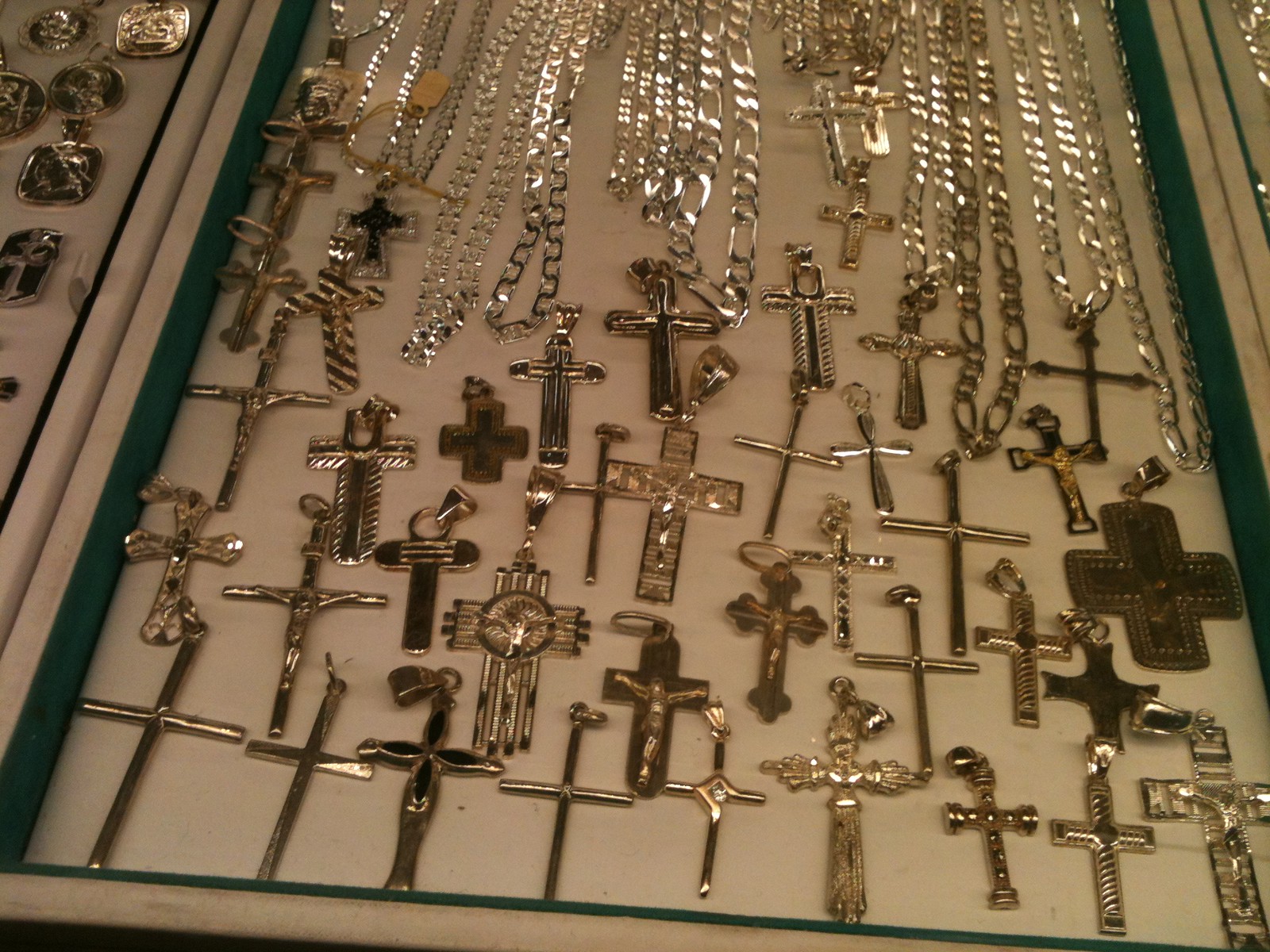The image is a horizontal rectangle photograph featuring a display case full of gold and silver crosses and crucifixes. The background of the display is white, framed with green edging on the sides. The cream-colored display case, which is slightly raised and probably has a glass top, is adorned with green velvet around its sides. Inside, there are numerous gold crucifixes of varying sizes, shapes, and designs, some adorned with intricate patterns or depicting Jesus on the cross, while others are plain. Scattered among the crosses, there are a few brooches and pendants. Above the display, there are thick, gold chain-link necklaces, reminiscent of 80s-style medallions, that can be paired with the crucifixes. The display creates a visually striking and diverse collection of religious jewelry.